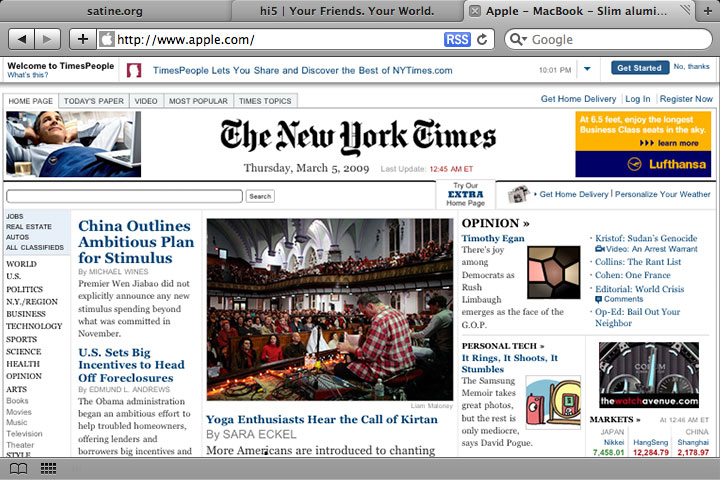This is a detailed visual description of a screenshot of The New York Times' online platform. At the top, the browser tabs are visible, showcasing three open tabs with titles: "Satine.org," "High Five Your Friends Your World," and "Apple MacBook Slim Aluminum." The search bar highlights a query for "Apple.com."

Below the browser, there's an announcement reading "Welcome to Times People," alongside a prompt that explains Times People allows users to share and discover the best of NewYorkTimes.com. The time displayed is 10:01 p.m., indicating that this page is being viewed on a computer. Users are given the option to get started or decline with "no thanks."

Prominently in the center, the New York Times logo is displayed in bold, elegant black text. The date is Thursday, March 5, 2009, with the latest update timestamped at 12:45 a.m. ET in red text.

On the left side of the image, there's a photo of a man lounging with a blanket and his hands behind his head. To the right, there is a colorful advertisement for Lithuania in gold and blue. Below this ad is an image resembling the interior of a packed church congregation. Amidst the crowd, a man in a plaid shirt appears to be sitting on the altar next to another man.

This page features several article headlines: "China Outlines Ambitious Plan for Stimulus," "U.S. Sets Big Incentives to Halt Foreclosures," and "Yoga Enthusiasts Hear the Call of Kirtan," which corresponds to the church-like image. Additionally, there are sections for Opinion, Personal Tech, and Markets.

On the left sidebar, a vertical menu allows readers to navigate through various topics such as Politics, World, U.S., Business, and Technology.